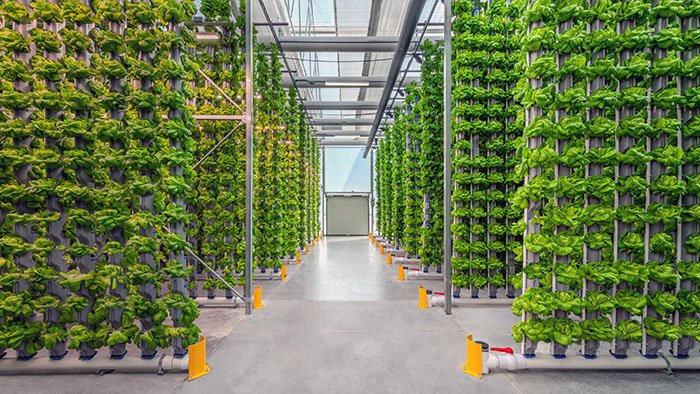This horizontally aligned, wide rectangular image depicts the interior of a large indoor nursery or greenhouse with a light blue backdrop. The building features a see-through ceiling made of clear plastic or glass, supported by gray pipes that likely assist in water transportation. Running down the center aisle are rows of short, green plants situated on narrow platforms or gray rods, which extend vertically and hold multiple tiers of plants, creating the impression of a vertical farm or library-like setup. 

The floor is a grayish marbled tile, and each section of plant rows is fronted by yellow plastic coverings or signs, which help differentiate the sections. There are also white pipes near the base of these rows, possibly involved in the irrigation system, transporting water upwards to the plants. Red valves can be seen at the ends of the containers, and various headlamps are installed at the top of the structure, providing necessary lighting for the plants.